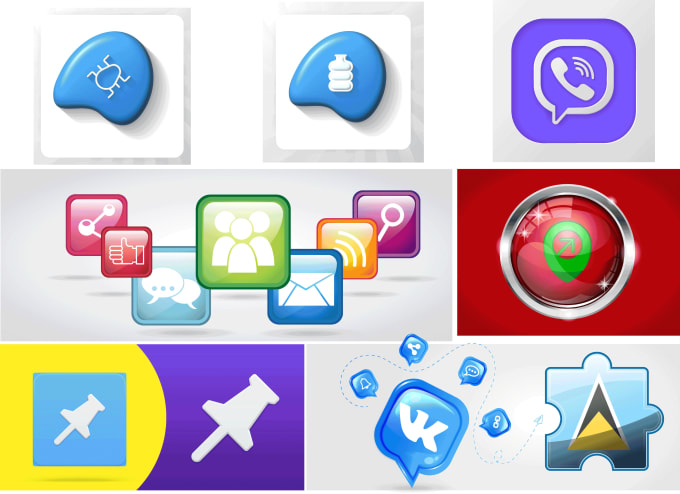The image is a rectangular, grid-like composition approximately six inches wide and four inches high, showcasing a collection of modern digital icons often seen on smartphones or tablets. The icons are diverse in color, featuring shades of red, green, purple, blue, yellow, and gold. The image is divided into thirds:

**Top Third:** It contains three main icons:
- **Left:** A white background with a gray border, featuring a blue guitar-pick shape with a white bug icon.
- **Center:** A similar layout showcasing a white icon resembling a three-layered water bottle.
- **Right:** A gray background with a blue square containing a traditional telephone icon inside a chat bubble.

**Middle Third:** This section features a long gray rectangle with various smaller colored squares:
- Icons include a thumbs up, chat bubble, three people, an envelope, sound waves, and a magnifying glass. 
- Right of center, there's a distinctive red square with a red circle, silver outline, and a green arrow inside.

**Bottom Third:** Consists of two main sections:
- **Left:** A yellow background with a blue circle containing a white thumbtack, adjacent to a purple background with another white thumbtack.
- **Right:** A gray background with a blue chat bubble featuring the letters "VK," accompanied by smaller blue chat bubbles, and a puzzle piece with a black and yellow triangle.

The overall aesthetic is clean and modern, characteristic of icons from stock image websites or app interfaces, with each section containing numerous icons that vary widely in design and function, from utilities like pushpins and telephones to social media symbols and more abstract graphics.